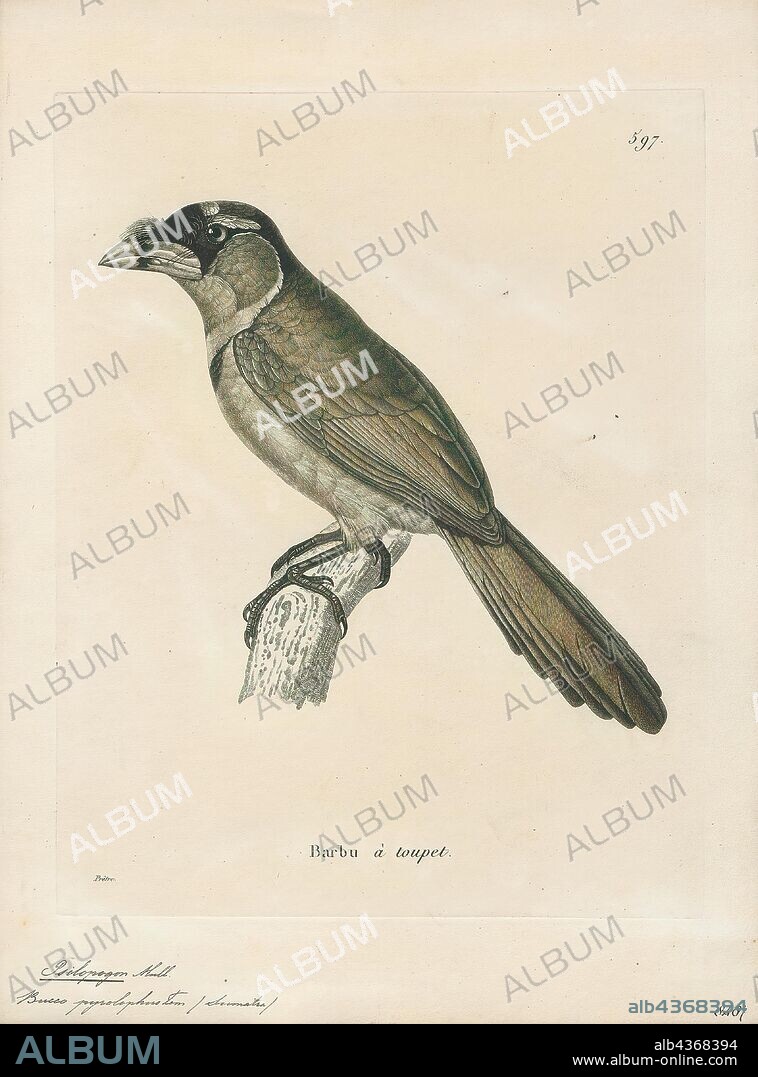This detailed and monochrome pencil illustration depicts a bird perched on a small, abruptly cut branch segment. The paper background is a medium tan-gray color. The bird, positioned to face the left, features a predominantly black head with a striking white area just above its eye, creating an almost eyebrow-like effect. Its beak is white, and its wings and tail are dark, with subtle shades of brown. The bird's belly is white, and its claws grip the branch firmly.

The illustration is overlaid with a diagonal watermark alternating in black and white text, stating "album." Additional text includes the words "barbu a trup" near the bottom, and very small cursive writing difficult to discern. The page number "597" is located at the top right. The bottom of the image includes a logo for "album" on the left and the website "www.album-online.com" on the right. A code number, ALB 4368394, is visible on both the image and an accompanying banner.